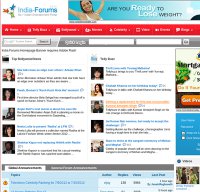The image is a screenshot of a webpage that is unfortunately blurry and hard to read. In the top left corner, there's text that reads "In Your Forums." Positioned to the right of this text is an image of a woman wearing a bikini top, accompanied by the phrase "Are you ready to lose weight?" Below this, there's a red rectangular menu that seems to activate a drop-down list when clicked, though the specific labels are indiscernible due to the image's blurriness.

Further down, there are two search bars: the one on the left is bordered in light gray, while the one on the right is bordered in dark gray. Below these search bars, a white area features ten cropped thumbnails arranged in two rows of five. There is an advertisement on the right side of this section, although it is partially cut off and cannot be fully viewed.

At the bottom of the image, an orange button labeled "Get" is visible. Below this button is a light blue box containing some text and what appears to be a couple of smaller boxes situated in the middle. The overall layout suggests this may be an interface related to health or exercise forums, given the contextual elements centered around weight loss.